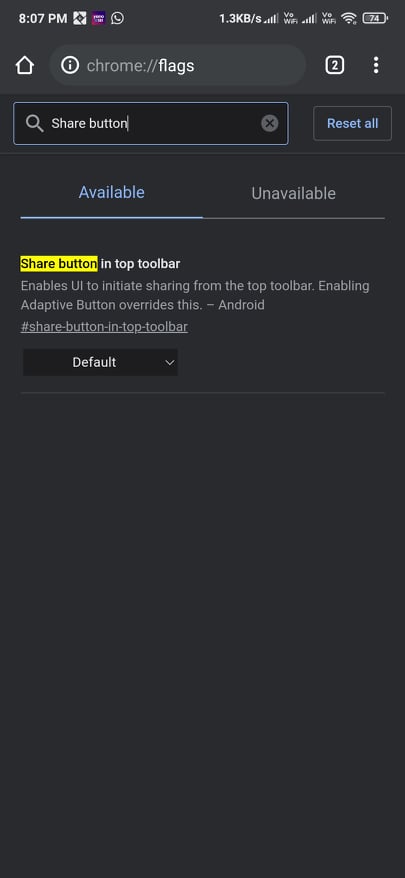Here's a detailed and cleaned-up caption for the image described:

"This screenshot displays a phone interface with a predominantly black background featuring white and light gray text, with some elements highlighted in blue. The time displayed is '8:07 PM' with a data size indication of '1.3 KB' and a symbol resembling a forward slash ('/S'). 

At the top of the screen is the URL bar, containing the URL 'chrome://flags'. Adjacent to the URL bar, a number '2' appears inside a white box next to a vertical ellipsis (three dots stacked vertically).

Below the URL bar is a search field labeled 'share button', followed by a blue button labeled 'Reset all'. Further down, the text reads 'available, unavailable', detailing options for features within the browser.

One listed feature is 'Share button in top toolbar,' which 'enables UI to initiate sharing from the top toolbar.' The text clarifies that 'enabling adaptive button overrides this' feature. Additionally, the description notes the feature's relevance under 'Android' and tags it with 'Hashtag share button in top toolbar default.'

Overall, the screenshot captures a detailed view of the browser settings interface, focusing on configurable features and their descriptions."